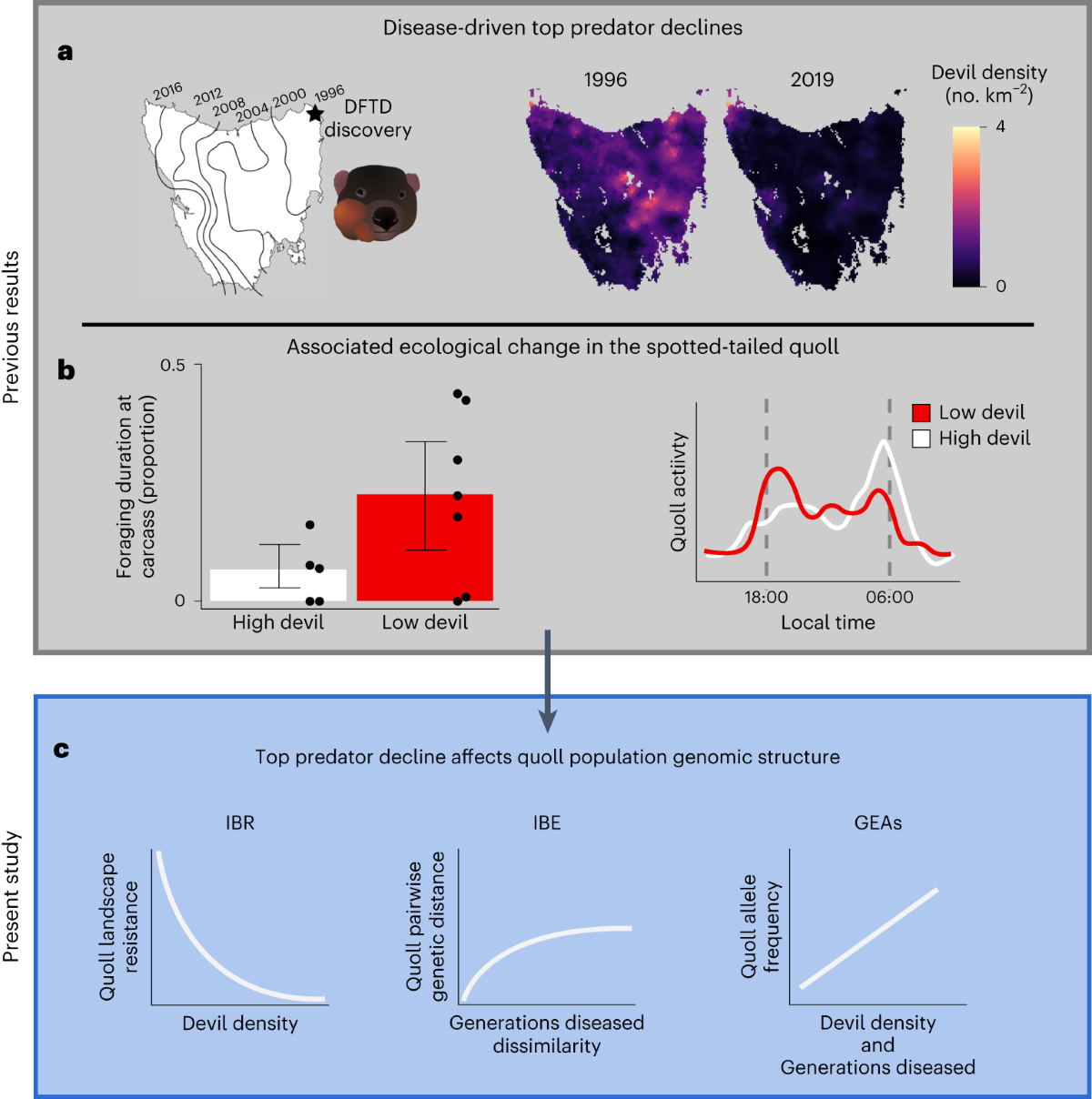The image is a detailed scientific chart illustrating the effects of disease-driven top predator declines, primarily focusing on Tasmanian devils and their impact on the ecosystem. The chart is divided into sections A, B, and C, each accompanied by graphs and heat maps.

Section A highlights the decline in Tasmanian devil populations from 1996 to 2019, showing devil densities over the years with heat maps that transition from dark purple (low density) to yellow (high density). It includes timestamps of significant years like the discovery of DFTD (Devil Facial Tumor Disease) and a timeline spanning from 1996 to 2016.

Section B details the associated ecological changes, particularly in the spotted-tailed quoll, with diagrams depicting foraging duration at carcasses.

Section C discusses the present study, showcasing how top predator decline affects the quoll population's genomic structure, with three graphs labeled IBR, IBE, and GEAS. The entire image is clear, well-lit, and brimming with intricate scientific data, effectively conveying the profound impact of predator declines on ecosystem dynamics.